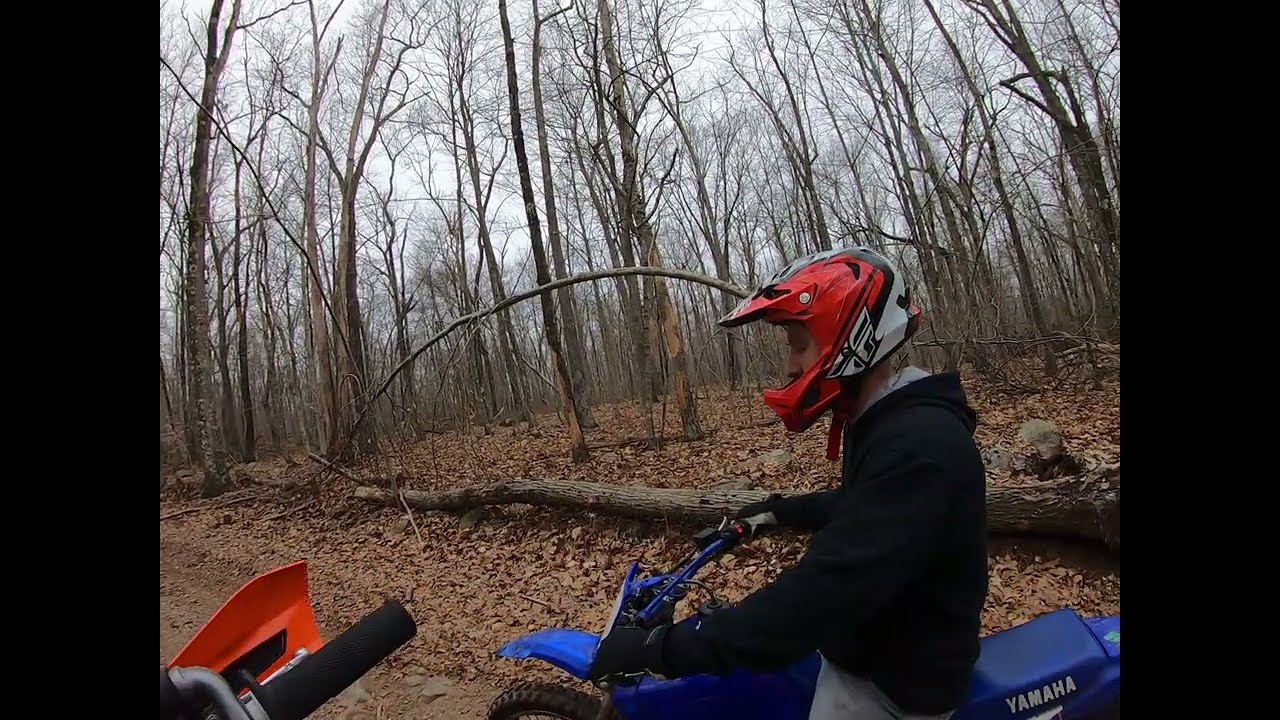The photograph captures an outdoor scene on a dirt road cutting through a barren forest, featuring two individuals on dirt bikes. One rider, centered prominently in the image, is atop a blue Yamaha dirt bike. They are clad in white pants and a black hoodie, with a red, white, and black helmet. The white "Yamaha" logo is clearly visible on the bike's blue seat. This rider appears to be gripping the handlebars, facing towards the left, with an overcast gray sky providing a somber background. 

In the bottom left corner, the handlebar of another dirt bike, likely belonging to the invisible photographer, is just visible. This bike appears to be red. Surrounding the dirt road, the ground is covered in brown leaves, and bare trees with fallen leaves further suggest the season is late fall. One notable feature in the landscape is a fallen log, positioned close to the edge of the path, adding to the rugged outdoor setting.